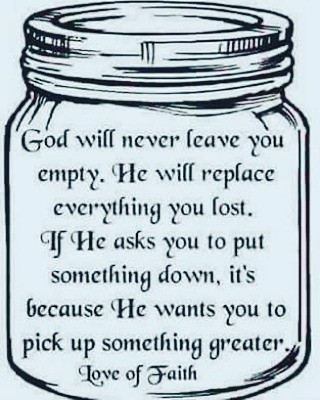The image features an intricately sketched mason jar with a screw-top lid, rendered in black ink with subtle shading at the top and bottom. Set against an eggshell blue background, the jar contains a meaningful quote in a somewhat fancy, italicized font, also in black ink. The text spans multiple centered lines inside the jar and reads: "God will never leave you empty. He will replace everything you lost. If he asks you to put something down, it's because he wants you to pick up something greater." At the bottom of the quote, it says, "Love of Faith." The whole design is enclosed in a vertical rectangular frame, making it suitable for home decor, social media graphics, or greeting cards.